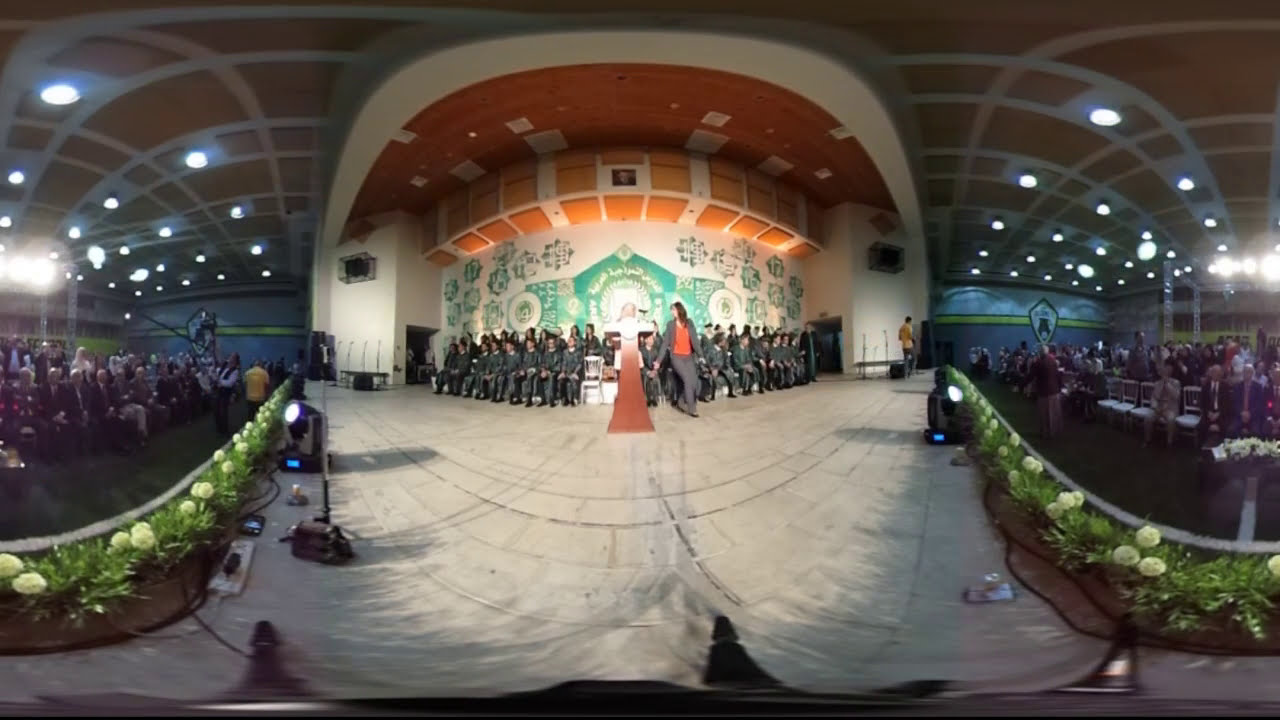This image captures a dynamic scene taking place in a large indoor auditorium with a stone or hard surface floor. At the center of the scene is an oval-shaped stage, where a graduation ceremony appears to be in progress. Seated in neat rows are numerous young individuals uniformly dressed in gray suits. They form a V-shape in front of a white curved backdrop, which features green designs and orange squares towards the top. At the front of the stage stands a podium, beside which is a person dressed in a gray suit and a red shirt, possibly making a speech or presentation. Surrounding the stage, which is festooned with white flowers and green plants, is a substantial audience both standing and seated on either side. Above, the ceiling features more intricate designs with white circles. The entire setting is decorated with a vibrant color palette, including black, white, off-white, green, orange, maroon, light blue, and purple. There are no visible text or banners in the image, which visually emphasizes the ceremonial and formal atmosphere of the event.